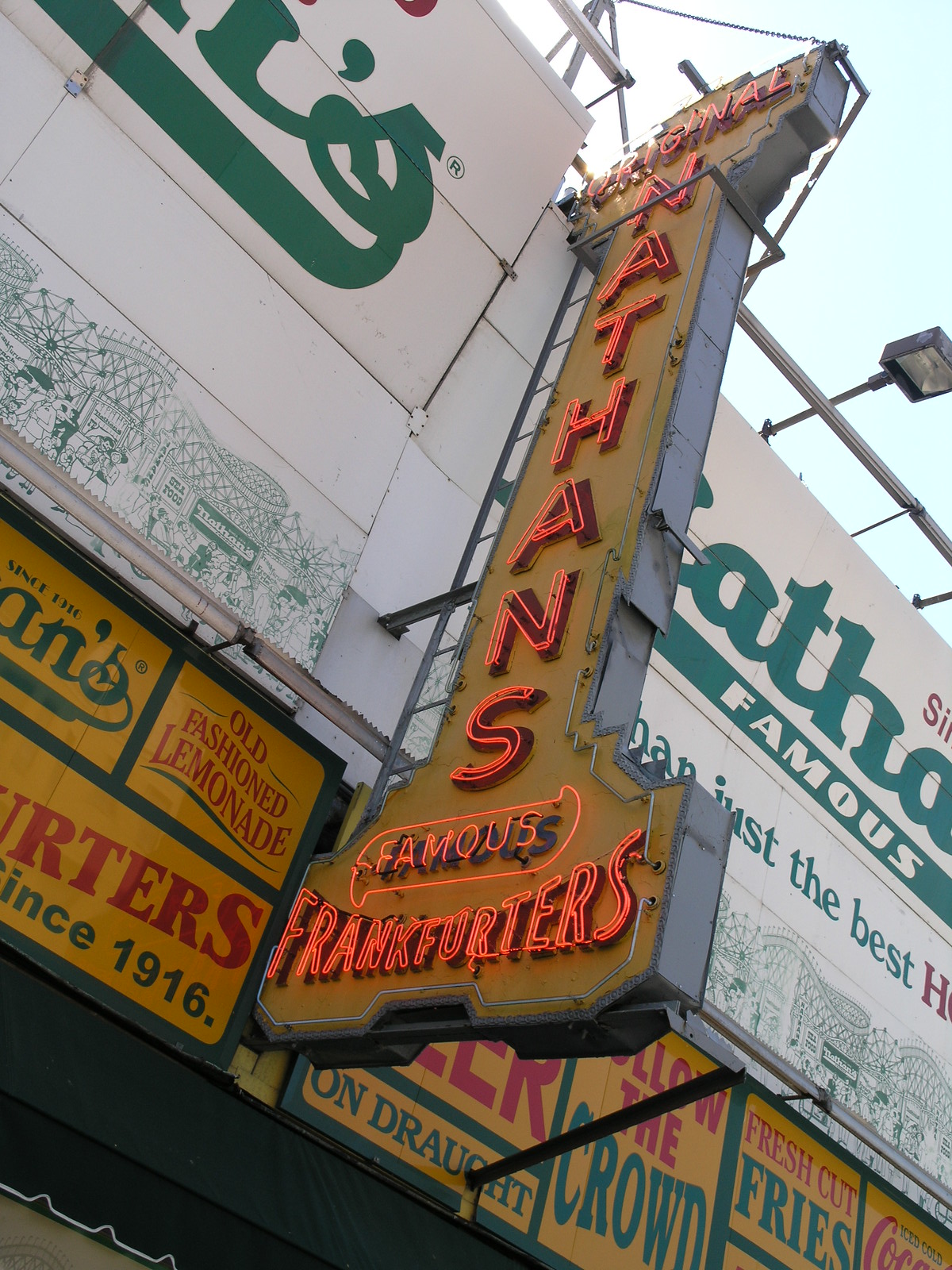This photograph captures an upward-looking view of the iconic storefront of Nathan's Famous Hot Dogs in Coney Island. Dominating the image is a tall, narrow neon sign jutting out from the side of the building. The sign, which has probably been a fixture for many years, features a yellow metal backdrop with white trim. The neon lights glow in a light orange hue, displaying "Original Nathan's" at the top, "Nathan's" vertically down the middle, and "Famous Frankfurters" at the bottom.

Above the storefront awning, there's a large billboard with a clean white background and the "Nathan's Famous" logo in green. The awning itself is adorned with various yellow placards advertising the establishment's offerings, such as old-fashioned lemonade, beer on draft, fresh-cut fries, and Coca-Cola. The combination of the historic neon sign and the vibrant promotional signs beneath it creates a nostalgic and lively atmosphere, reflecting Nathan's long-standing presence and popularity in New York.